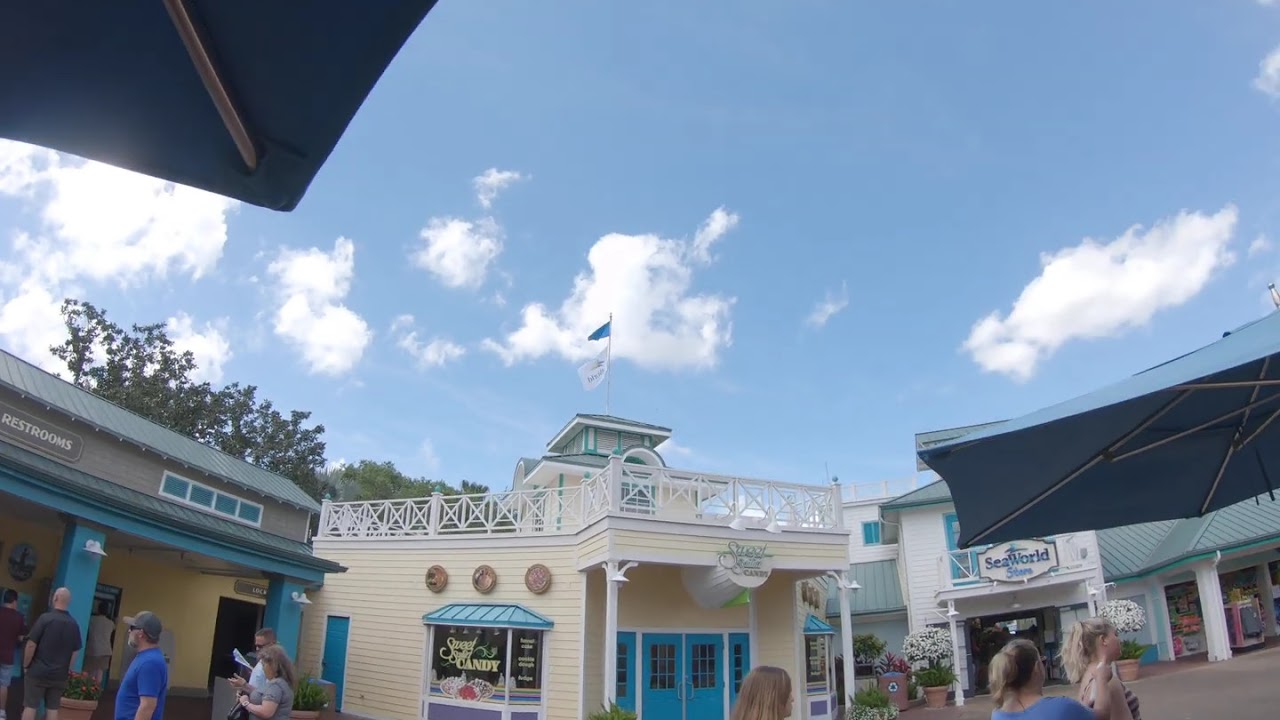The photograph depicts an outdoor scene at SeaWorld, reminiscent of a town square within an amusement park. The main focus is a brightly painted yellow sweet candy shop, adorned with white trim and turquoise blue doors. It has a charming, old-timey feel, enhanced by a small awning and a couple of flags—one white and one blue—on its roof. This candy shop, labeled "Sweet Select Candy," exudes a nostalgic charm, attractive to tourists. 

To the right of the candy shop, there is a SeaWorld Store with a teal rooftop and a sign displaying the words "SeaWorld Store." Its facade features off-white siding with mint green roofing, providing a coastal aesthetic. Pedestrians stroll about the area, adding a lively vibe. 

In the foreground, some large blue umbrellas and potted flowering plants contribute to the inviting atmosphere. On the left side of the image, a building marked "restrooms" is visible. The photograph, taken in the middle of a clear, partly cloudy day, captures a bustling, yet serene slice of SeaWorld's amusement park environment.